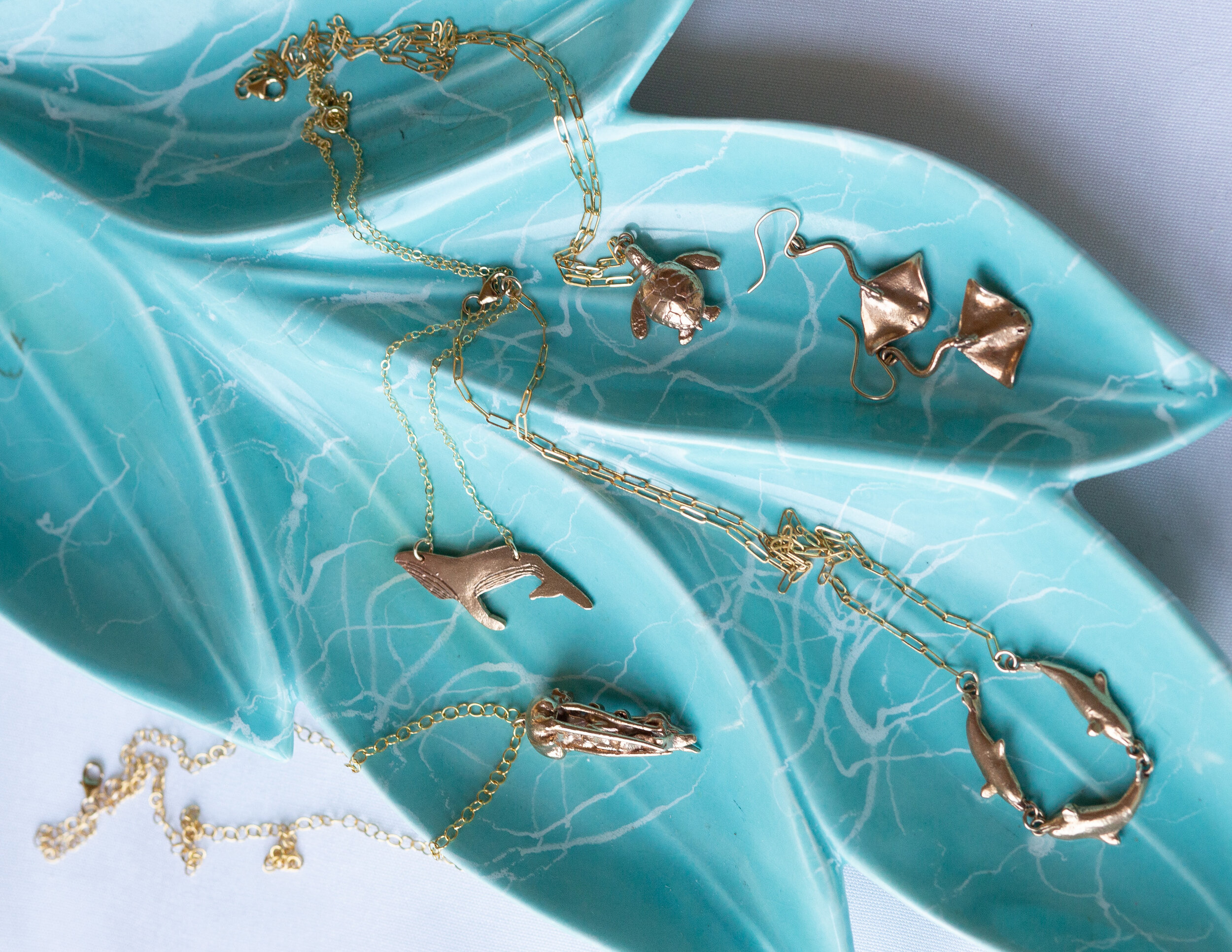This photograph captures a detailed view of a turquoise, leaf-shaped jewelry holder set on a white surface. The holder is intricately designed to mimic the natural form of a leaf, and it's adorned with white splashes that evoke an oceanic feel. Spread across the holder are various pieces of gold jewelry, all with a seaside theme. 

On the top right of the holder are two gold earrings shaped like stingrays. Just to the left of these earrings is a necklace featuring a gold turtle charm, and below this necklace is another adorned with a blue whale pendant. Towards the bottom right of the holder lies a necklace with three interconnected gold dolphin charms. Scattered among these are additional ocean-themed jewelry pieces, including a bracelet with a humpback whale pendant and other charms that are harder to identify. The overall arrangement of the jewelry enhances the seaside motif, beautifully complementing the ocean-like design of the blue tray.